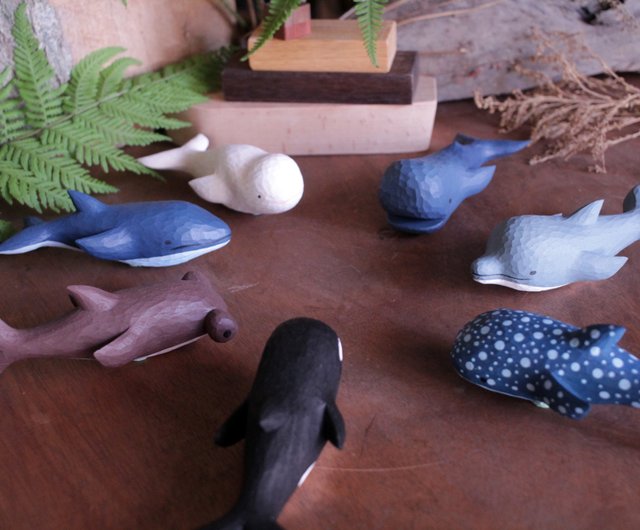This detailed image portrays a brown wooden table or counter with seven colorful and intricately painted marine figurines carefully arranged in a circle, their mouths pointing inward as if engaged in a silent gathering. Starting from the lower center and moving clockwise, the figurines include a black and white orca, a brown hammerhead shark, a blue and white whale, a white beluga, a blue whale with its mouth slightly open, a gray and white smiling dolphin, and a dark blue fish with light blue polka dots. Adding to the charm, the background includes a green leaf in the upper left corner, a brown branch in the upper right, and a small, stacked wooden boat-like structure towards the back, crafted from three rectangular blocks. This arrangement creates a balanced and visually engaging scene, with hints of nature accenting the table setup.